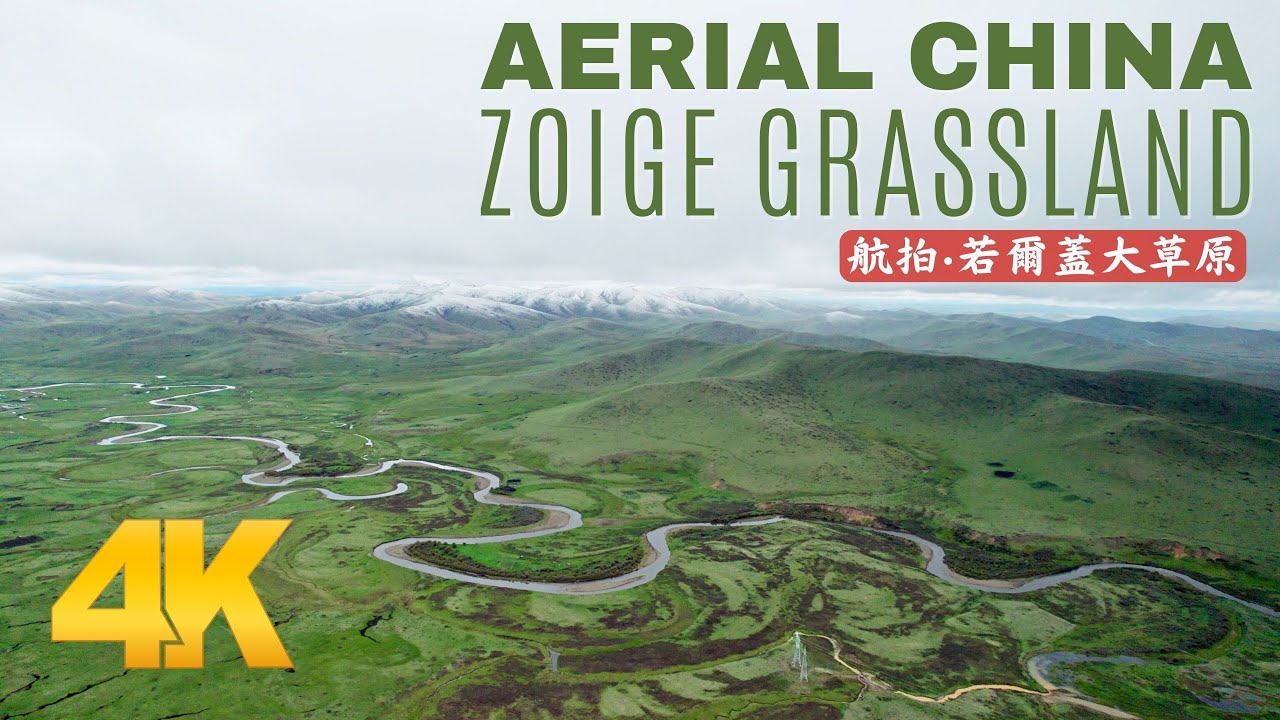This image is a scenic poster or screenshot showcasing the captivating landscape of Zoige Grassland in China, as advertised for a video or TV program titled "Aerial China." The lower half of the image features a vast green expanse through which a winding river snakes from the bottom right to the top left, forming intricate meanders across the valley. The left side of the river is characterized by flat grasslands interspersed with clumps of dirt, while the right side showcases hilly, densely vegetated plains. In the background, a majestic mountain range with snow-capped peaks stretches across the top center and right, under a thick, gray, overcast sky. The top right corner of the image contains the text "Aerial China" in green letters, with "ZOIGE Grassland" in black letters beneath it, accompanied by a red bar featuring white Chinese characters. The bottom left corner prominently displays "4K" in large yellow letters, indicating the high-resolution quality of the visual content.